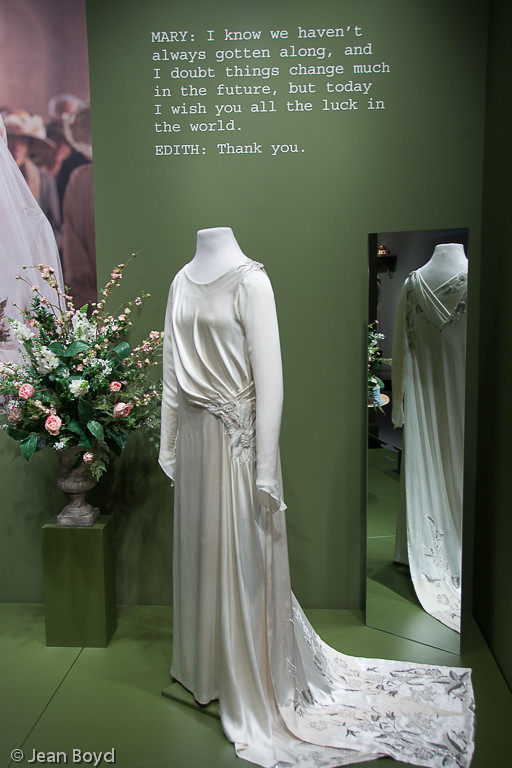This image features an elegant display for a white wedding dress adorned with a long, flowing cape that beautifully transitions into a floral print featuring birds and an overall happy scene. The dress, set on a headless white mannequin, showcases intricate embroidery of white flowers around the hips and the bottom. The mannequin is situated in a meticulously curated green-themed setting.

In the left foreground, a square green stand holds a tasteful flower arrangement consisting of pink, white, and green foliage, adding a touch of natural beauty to the scene. The backdrop of the display is a green wall featuring a heartfelt message: "Mary, I know we haven't always gotten along and I doubt things change much in the future, but today I wish you all the luck in the world, Edith. Thank you." This message suggests a poignant exchange between two individuals, Mary and Edith.

Adjacent to the dress, there's a mirror that allows viewers to appreciate the intricate details of the cape's back. The scene also includes a subtle, possibly purple-sepia toned area to the left, hinting at the presence of obscured figures, likely a picture of women. In the bottom left corner of the image, the text "copyright Gene Boyd" is visible, crediting the creator of this vivid and detailed display.